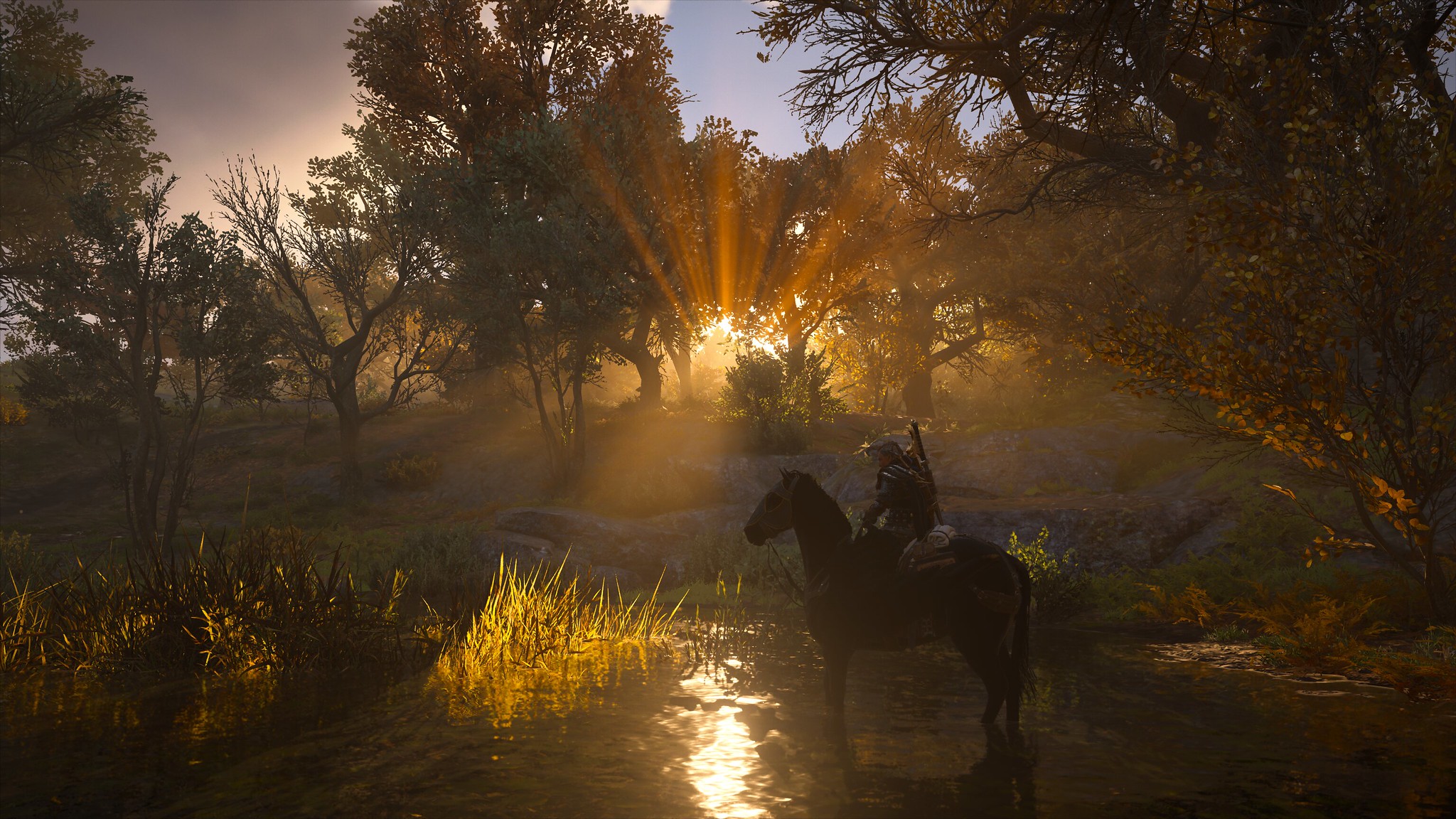A rider is prominently positioned on a horse in the foreground, with a rifle slung over their back. The ground beneath them is wet and reflective, possibly indicating a recent rain. In the background, a barren tree stretches its leafless branches skyward. The ground around the tree consists of dry grass interspersed with puddles. Sunlight filters through the tree branches, creating a glow that enhances the scene. To the side, a bush with some grass adds to the natural setting. The sky above is predominantly blue, with a grey cloud situated in the top left corner. Near the edge of the scene, there is foliage from another tree, adding depth to the composition.